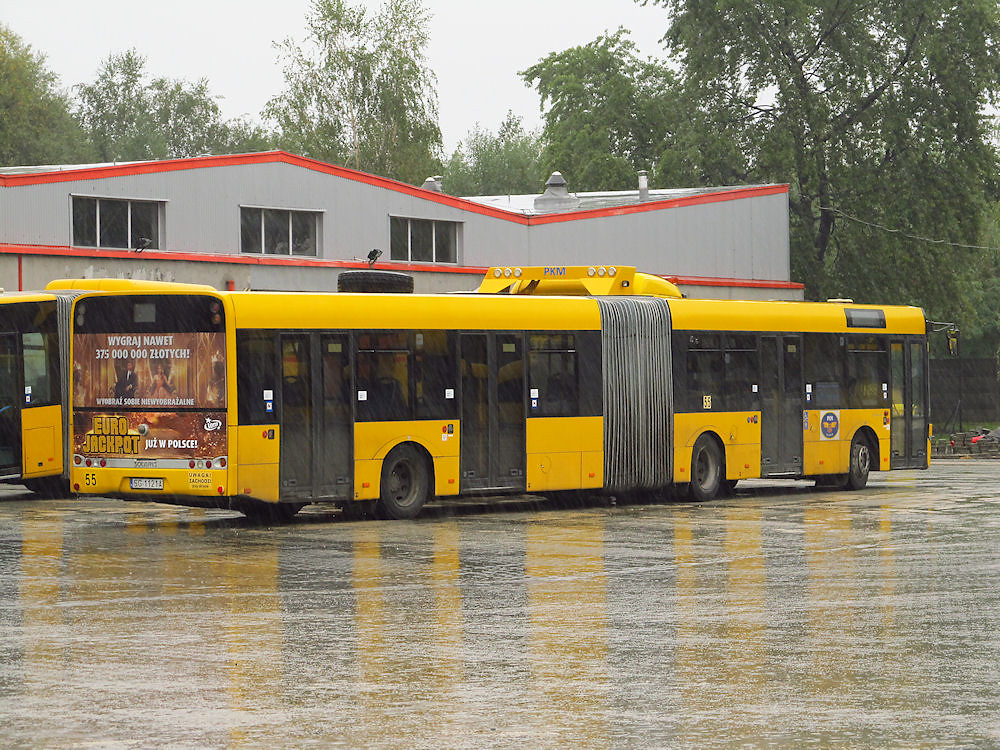This image captures a long, articulated bus with a distinct accordion-style connector in the center, resembling two school buses joined together. The yellow bus has six tires across three axles, and its design allows passengers to walk from front to back seamlessly. The bus is parked in a wet, reflective parking lot in front of a low, flat-roofed, gray building with orange trim and three second-story windows. The advertisement on the rear of the bus promotes "Eurojackpot," suggesting the photo is taken in a European country. Surrounding the area are green trees, hinting at a forested backdrop, and the overcast sky contributes to the rainy, shiny appearance of the scene.